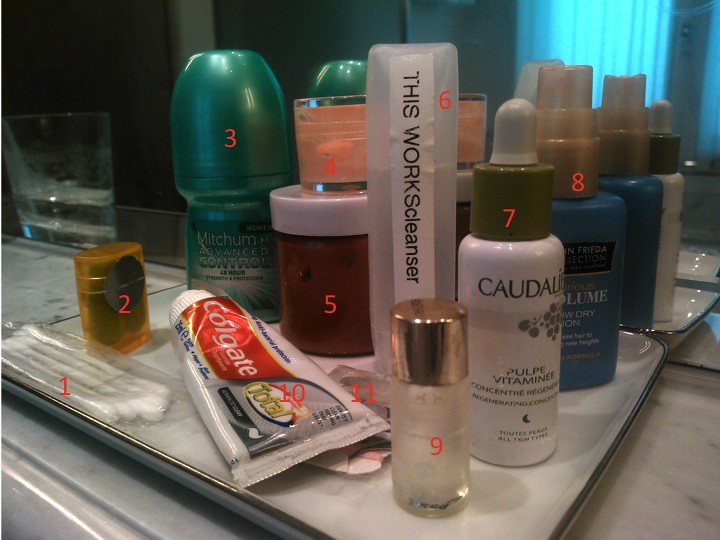The bathroom counter is adorned with an array of hygiene and beauty products, each meticulously labeled with a distinctive red number. At the center, prominently displayed, is a tube of Colgate Total toothpaste, identifiable by its distinctive red label emblazoned with "Colgate Total" and marked as number 10.

1. A package of cotton swabs sits on one end, essential for various grooming tasks.
2. Nearby is a small, elegant gold bottle, which appears to contain perfume.
3. A green bottle of Mitchum Advanced Control deodorant, essential for daily freshness, is marked next.
4. A charming pink candle, adding a touch of coziness to the space.
5. A jar containing a mysterious brown substance, sealed with a white lid.
6. A tall white bottle boldly labeled "This Works Cleaner," likely a cleaning product for the bathroom.
7. Another white bottle featuring an olive-colored lid with the label "Pupil Vitamin," presumably a wellness supplement.
8. A blue bottle with a brown lid, its label unreadable, adding to the intrigue of this collection.
9. Lastly, a small white bottle with a gold screw-top lid, devoid of a label, leaving its contents a mystery.

This detailed arrangement of personal care items reflects a well-organized and comprehensive approach to hygiene and beauty.